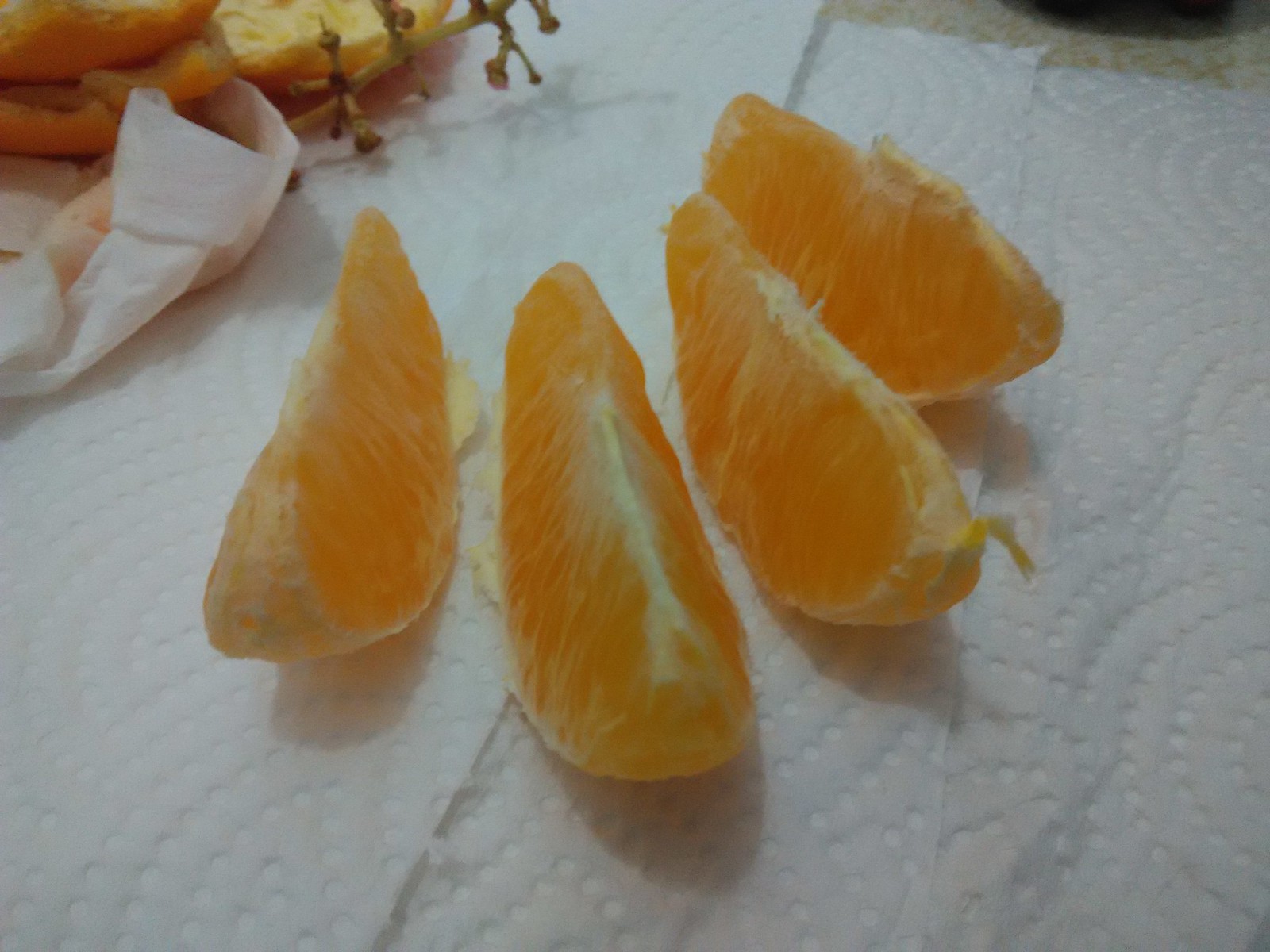The photograph features four bright orange slices carefully balanced upright on their sides, positioned on a white paper towel that covers the surface of a table. Each slice displays a bit of the inner white peel still clinging to it. To the upper left of the orange slices, there is a yellow grape stem, now bare after the grapes have been removed. Additionally, remnants of the orange rind are visible in the corner. The paper towel not only serves as a base for the orange slices but also partially covers the edge of a dark-colored bowl or cup and a piece of white cloth.